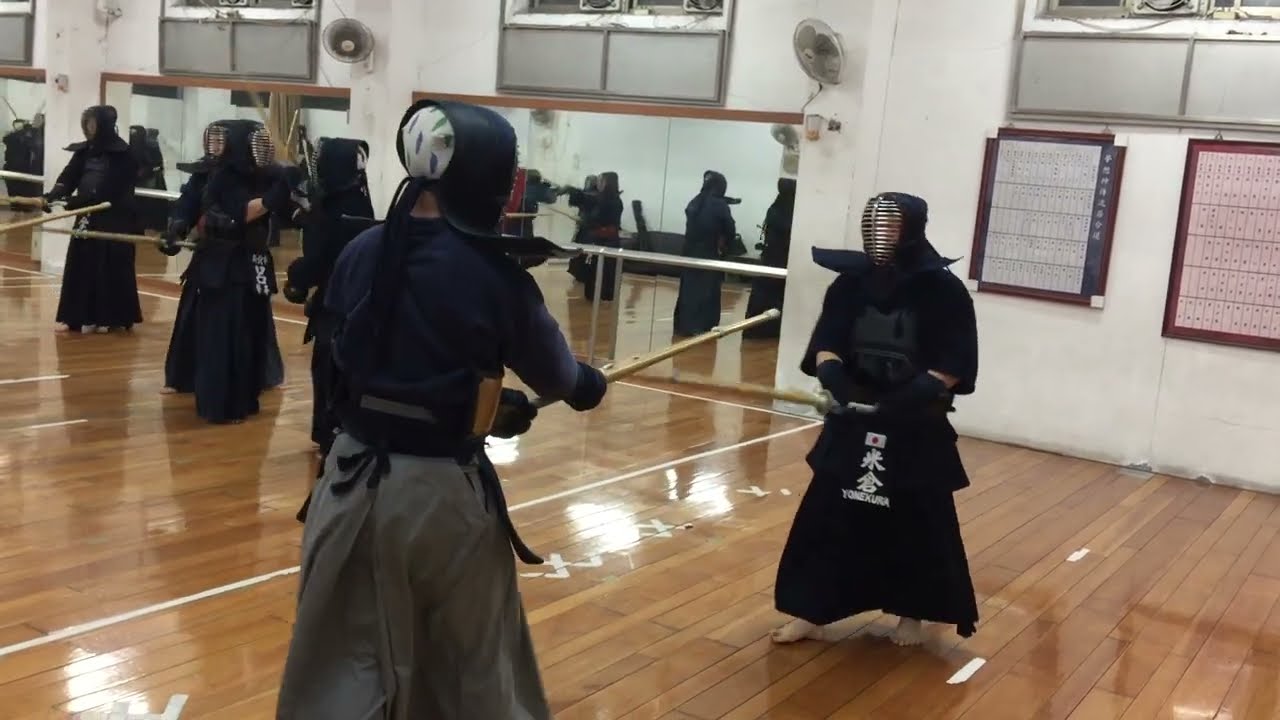This image captures an indoor kendo sparring session within a spacious studio characterized by its polished, shiny wooden floor and white walls. The focal point is two practitioners in the foreground, positioned centrally. The individual facing the camera is dressed in a black robe adorned with white writing and symbols, a black headscarf, black gloves, and a metal kendo mask. Opposite them, with their back to the camera, stands another combatant in a black top and gray bottom, also wearing a black headpiece and possibly a metal mask, and holding a metal pole towards their opponent. The studio features tall mirrors on the left wall, reflecting additional practitioners similarly attired. Ceiling fans and wall-mounted fans are visibly in place, maintaining the room's airflow. Various pieces of artwork and charts embellish the background, adding cultural context to the martial arts setting.